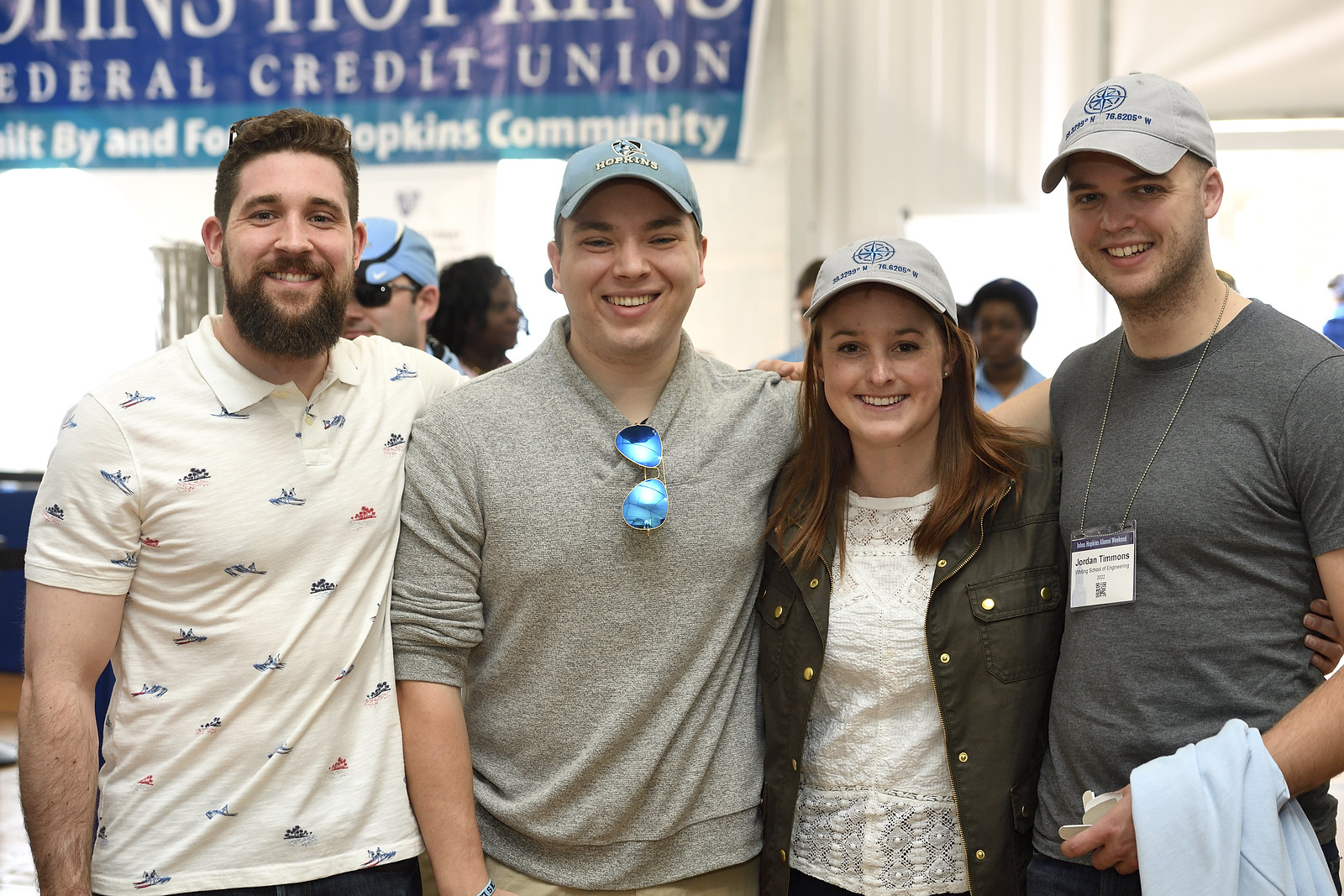This full-color photograph features four young individuals, likely in their late 20s or early 30s, posing closely together with their arms around each other, smiling and looking very happy. The scene unfolds indoors during daytime, possibly at the grand opening of a credit union, as suggested by the presence of a banner in the background that reads, "Federal Credit Union built by and for Hopkins Community." There are several people in the background, presumably employees, given their blue attire.

From left to right, the first individual is a man with dark hair and a beard, wearing a white polo shirt decorated with images of boats, and sporting sunglasses perched atop his head. Next to him is another man wearing a light blue Hopkins baseball cap, and a gray sweatshirt with the sleeves pushed up, with blue reflective aviator glasses hanging from the neck. Beside him stands a woman in a white lace top and a dark jacket adorned with silver buttons; she has reddish-brown hair cascading past her shoulders and is also wearing a gray baseball cap with a compass logo and coordinates. The man on the far right is dressed in a dark heather gray shirt and has a lanyard with a name tag around his neck. He is notably holding what appears to be a shirt or towel over his left arm and shares the same cap as the woman beside him.

Overall, this candid group shot captures a moment of camaraderie and celebration among friends or colleagues, unified by their shared attire and joyful expressions.